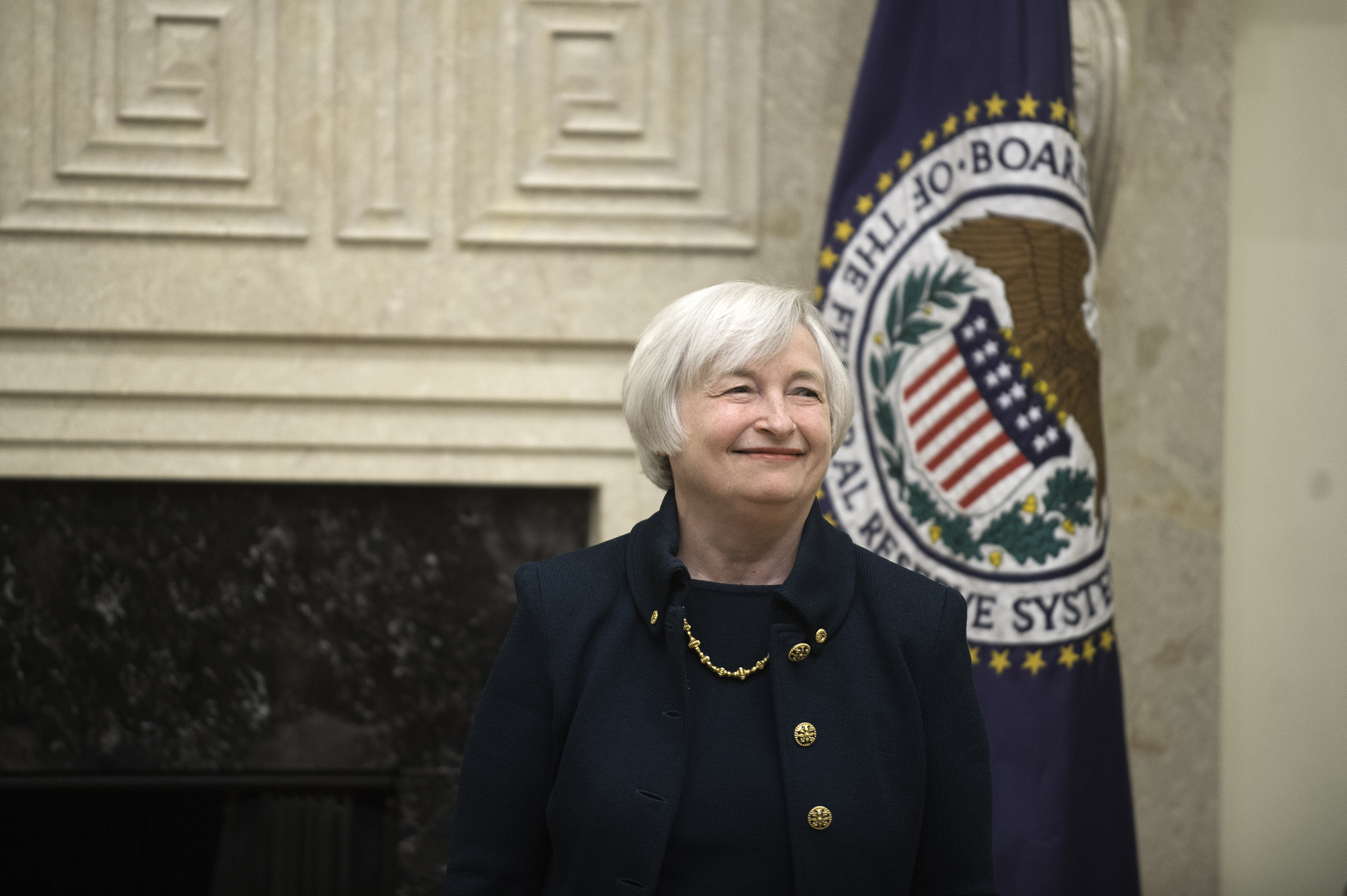This detailed photo captures Janet Yellen, the Secretary of the Treasury, standing indoors, likely within a government building. Yellen, who is smiling pleasantly, has short, completely white hair styled in a bob cut. She is dressed in a navy blue suit jacket adorned with three prominent gold buttons on the left side, paired with a matching navy blue shirt and a gold necklace that adds a touch of elegance. Behind her, on the right side of the image, is the Federal Reserve System flag, characterized by a blue field, an eagle, a shield with red, white and blue stripes, stars, and olive branches. To the left, a gray marble fireplace is visible, complete with a metal screen. The background includes a white wall with molding, adding to the official ambiance of the setting.